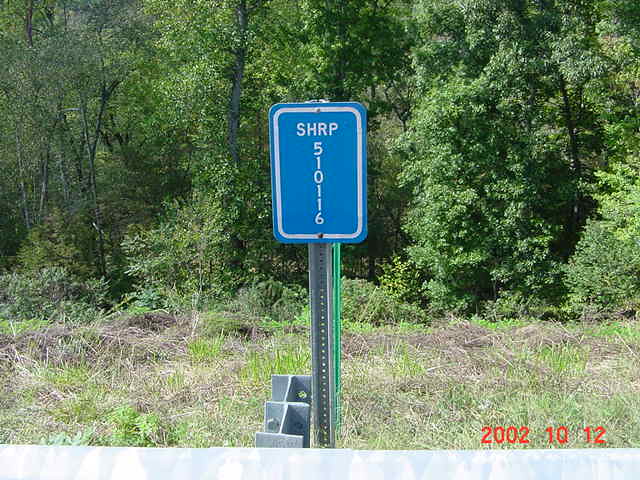In this image, a small gray pole supports a blue street sign amidst a densely forested area. The vibrant green foliage dominates the background, creating a lush natural setting. The blue sign, framed with a white border, prominently displays the capital letters "SHRP" in white, with the number "510116" printed horizontally below. Both elements are clearly distinguished against the blue background. In the bottom right corner, the date "2002-10-12" is visible, suggesting when the photo was taken. To the left of the gray pole, two gray structures resembling bricks appear to be stabilizing the sign, contributing to the detailed composition of the scene. The ground in the foreground is covered with light green to yellowish grass, adding a patch of contrasting color to the image.